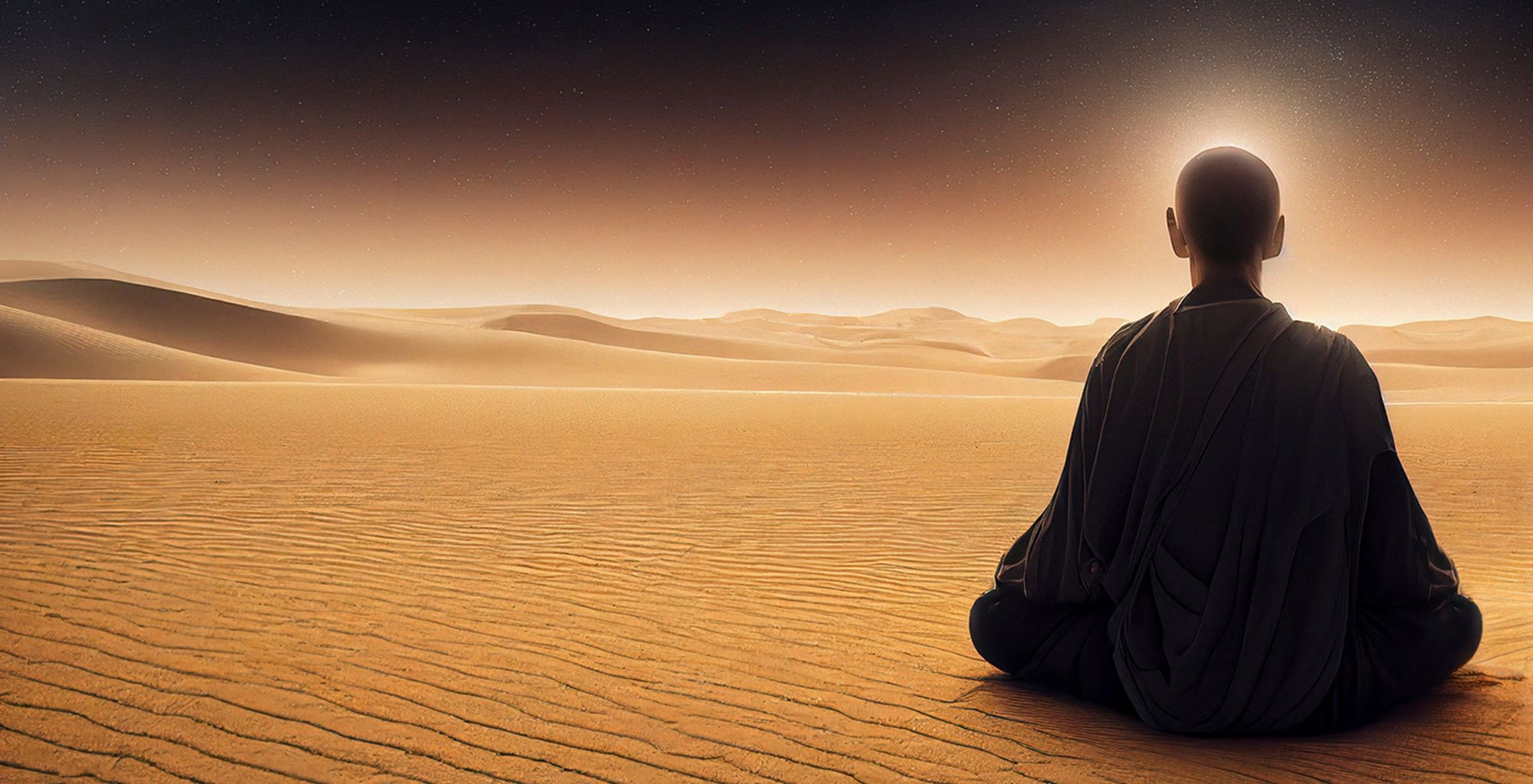In this striking, mystic-styled photograph, a solitary human figure, resembling a Buddhist monk, sits cross-legged in a meditative lotus position on the rippling sands of a vast desert expanse. Viewed from behind, the figure's bald head and close-cropped hair are illuminated by a halo-like glow that harmonizes with the light emanating from the horizon. Draped in a long robe, possibly with a hood, the monk's dark clothing contrasts with the vibrant landscape. The desert extends into the distance with undulating sand dunes bathed in an ethereal light that transitions from a bright yellow near the horizon to deep oranges and browns, eventually blending into a dark blue sky overhead. This serene and contemplative image captures the tranquil essence of meditation amidst the endless, sun-drenched sands.